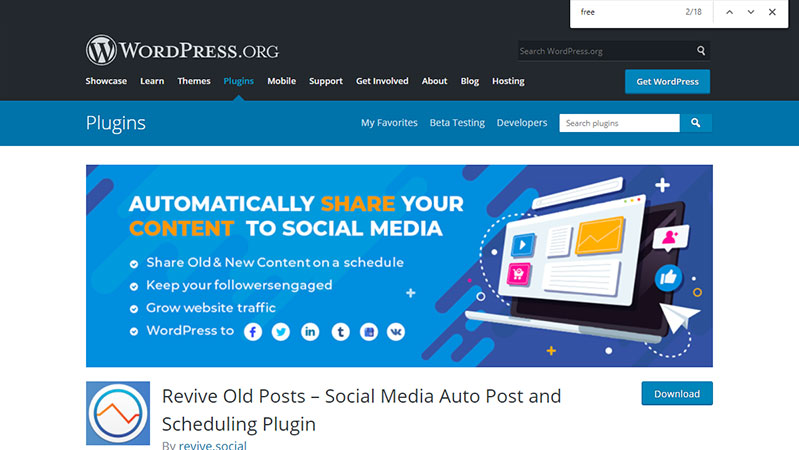The image depicts the homepage of wordpress.org. The top navigation bar features links to key sections: "Showcase," "Learn," "Themes," "Plugins," "Mobile," "Support," "Get Involved," "About," "Blog," and "Hosting." Prominently displayed is a button labeled "Get WordPress." A blue-highlighted section labeled "Written Plugins" is open, with other tabs like "My Favorites," "Beta Testing," "Developers," and a search bar nearby.

An advertisement on the page promotes a plugin that automatically shares content to social media platforms like Facebook, Twitter, LinkedIn, and Tumblr, emphasizing its ability to share both new and old content on a schedule to keep followers engaged and grow website traffic.

Adjacent to the ad is a graphic image, accompanied by text advertising the "Revive Old Posts" plugin, which focuses on social media automation and post scheduling. The advertisement concludes with a "Download" prompt on the side.